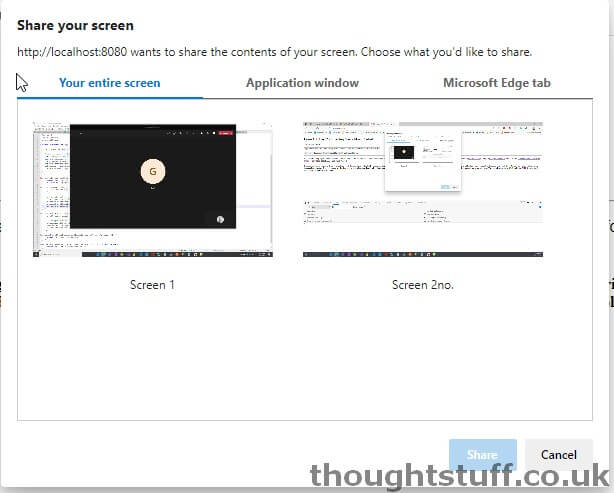Here is a cleaned-up and detailed caption for the image described:

---

Screenshot of a screen-sharing prompt with a white background. At the top, in black font, it reads "Share your screen." Below that, the text "http://localhost:8080 wants to share the contents of your screen. Choose what you'd like to share" is displayed. Beneath this message, there is a menu offering three sharing options: "Your entire screen," "Application window," and "Microsoft Edge tab," with "Your entire screen" selected. 

The interface shows two screen previews:
- **Screen 1:** Displays a black window with a white circle in the center containing the letter "G."
- **Screen 2:** Appears to show an image of a check or a scanned document.

At the bottom of this prompt, two buttons are visible:
- A blue rectangle with white text that reads "Share."
- A gray rectangle with black text that reads "Cancel."

Lastly, at the very bottom, the text "thoughtstuff.co.uk" is written in gray font. The entire screenshot is bordered with gray lines.